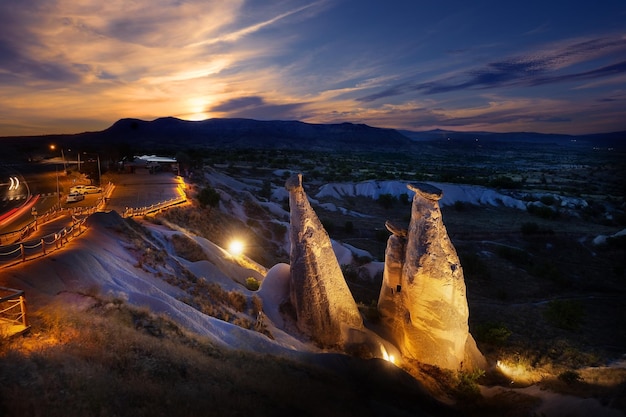The photograph captures an enchanting twilight landscape, possibly taken just after sunset or just before sunrise, characterized by its captivating interplay of light and shadow. Prominent in the background are dark, silhouetted mountains, with a faint hint of snow in certain spots. A delicate, blue twilight sky stretches above, streaked with ephemeral clouds, while the sun peeks shyly from behind the mountain line, casting a soft, ambient glow.

In the midground, there are two tall, skinny plateaus with flat rock tops, dramatically illuminated by artificial lights. These rock formations are situated on a grassy slope, also adorned with additional smaller rocks. To the left, a well-lit road meanders through the scenery, flanked by fences and a parking lot where a few cars are blurred in motion, their headlights creating a dynamic, streaking effect in the dim light. The road, having two sides for bi-directional traffic, features a red traffic light currently halting a trio of vehicles. Faint city lights twinkle in the distant background, contributing to the serene, yet slightly surreal atmosphere of this beautifully composed landscape shot.